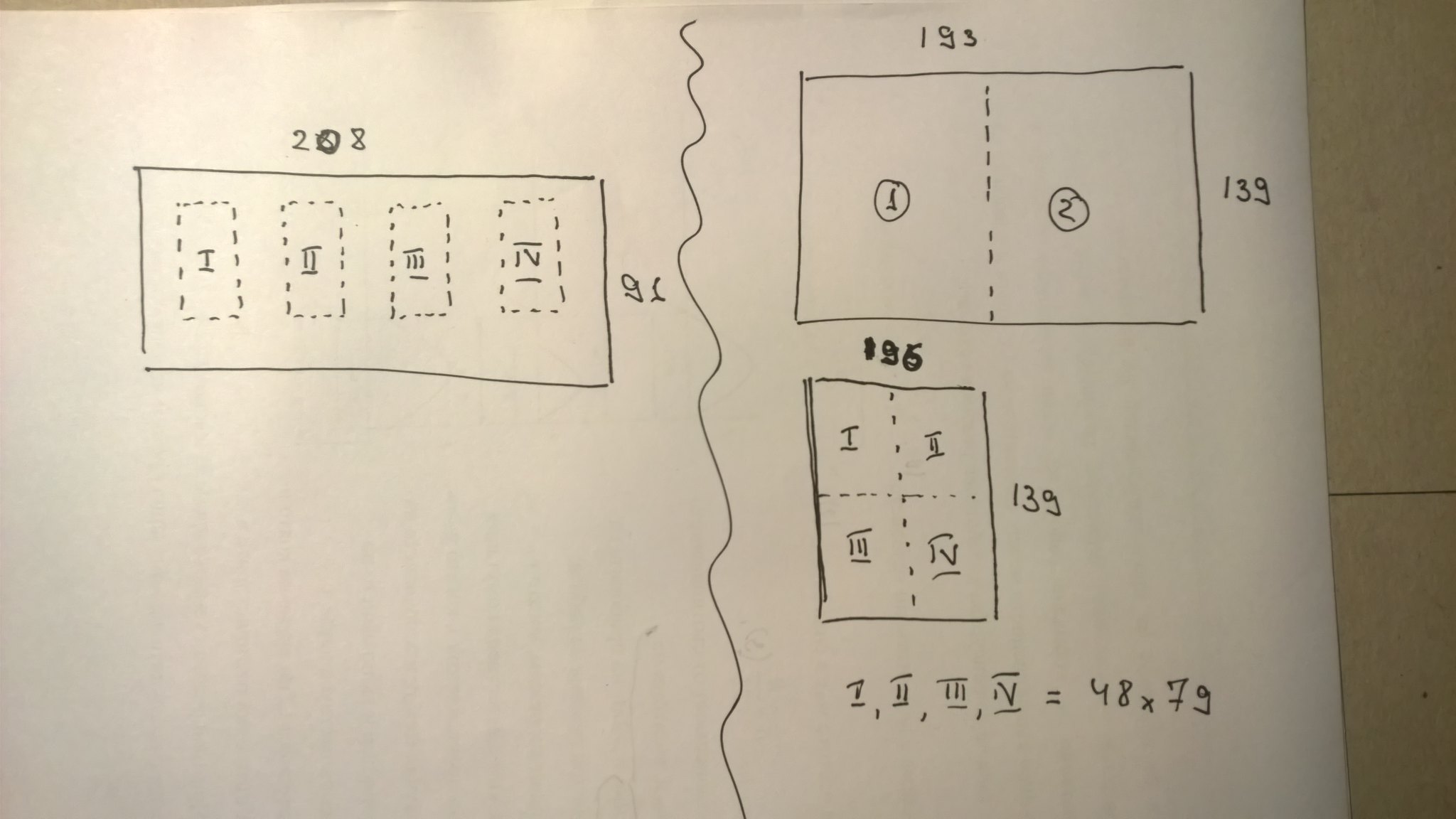The image depicts a hand-drawn map on a white piece of paper, viewed from a top-down perspective. The map illustrates four distinct building shapes. 

1. **Left Building**: 
   - This structure is divided into four units, each labeled with Roman numerals I, II, III, and IV.
   - It is enclosed within a dashed rectangle.
   - The numbers "208" and "91" are annotated above this building, likely indicating dimensions (208 by 91).

2. **Central Divider**:
   - A squiggly line runs vertically, separating the left and right sections of the map.

3. **Right Building**: 
   - Another rectangular box is present, containing two sections labeled with numbers "1" and "2" inside circles.
   - These two sections are divided by a dashed line.
   - Above this box, the number "193" is written, and "139" is annotated on the right side.

4. **Lower Section**:
   - Below the right building, another structure is represented with four units, each also labeled as I, II, III, and IV, and separated by dashed lines.
   - The number "196" is written on top of one of the units, and "139" is inscribed to the right.
   - Further below, an additional notation lists the Roman numerals I, II, III, and IV, followed by "48x79", indicating possible dimensions (48 by 79).